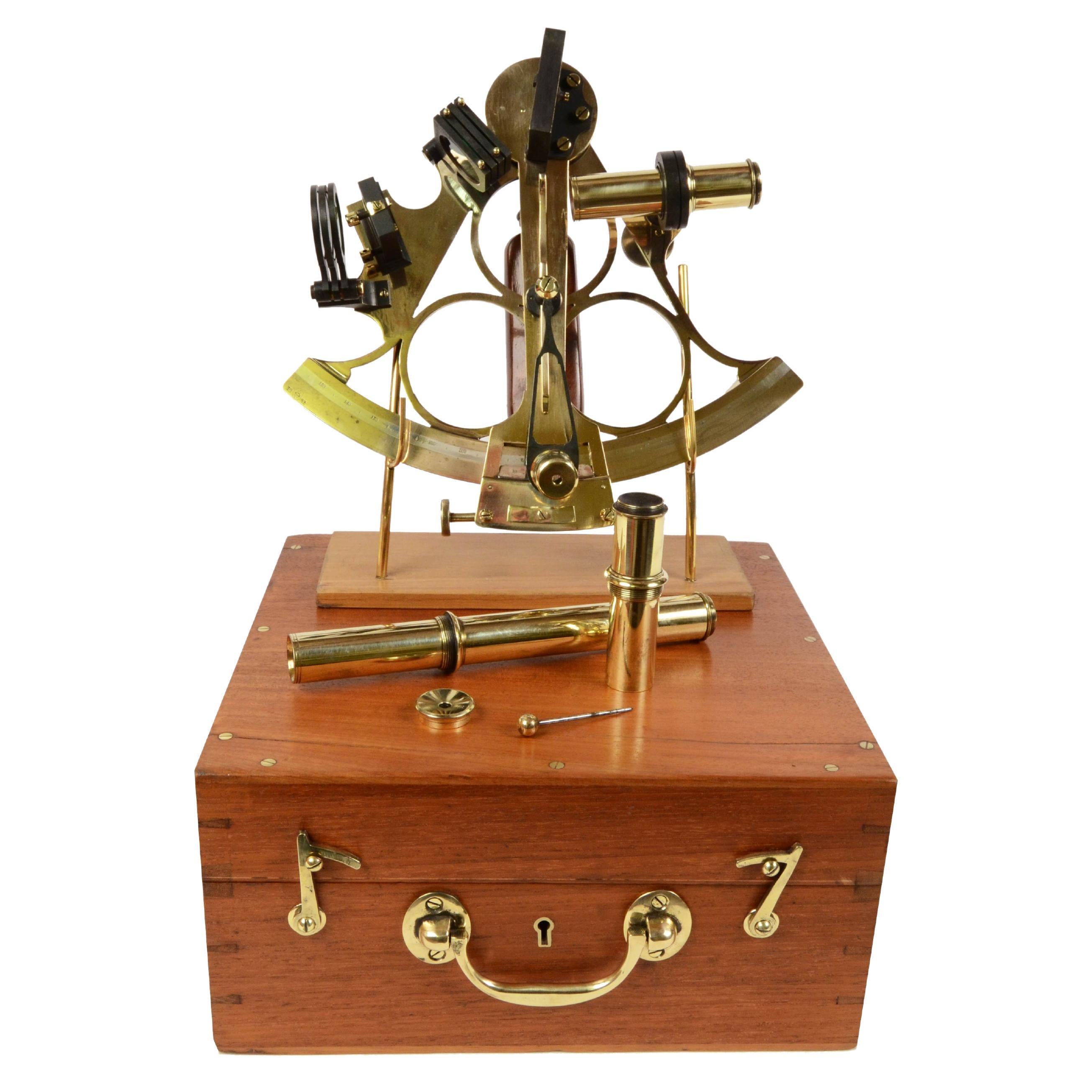The image showcases a historical navigational device known as a sextant, mounted on a wooden plank. This intricately designed instrument features two posts that potentially serve as balance points during use. Positioned in front of the device are two long, tubular lenses, distinguished by their gold finish. These lenses rest atop a squared wooden box equipped with peg grooved sides, indicative of its age.

The wooden box itself is quite detailed, with gold handles and latches on either side of a central gold handle, complemented by a keyhole resembling that for a skeleton key, adding a touch of elegance and security to the storage container. The box also features two gold locks on its front side, further emphasizing its function to safeguard the valuable sextant inside.

The sextant, traditionally used by sea captains to determine their location at sea by measuring celestial objects, has a rounded, curved base with measurement markers. The device includes a small viewing tube on the right-hand side and multiple magnifying glasses on the left, enabling precise alignment with the stars to navigate during nighttime voyages.